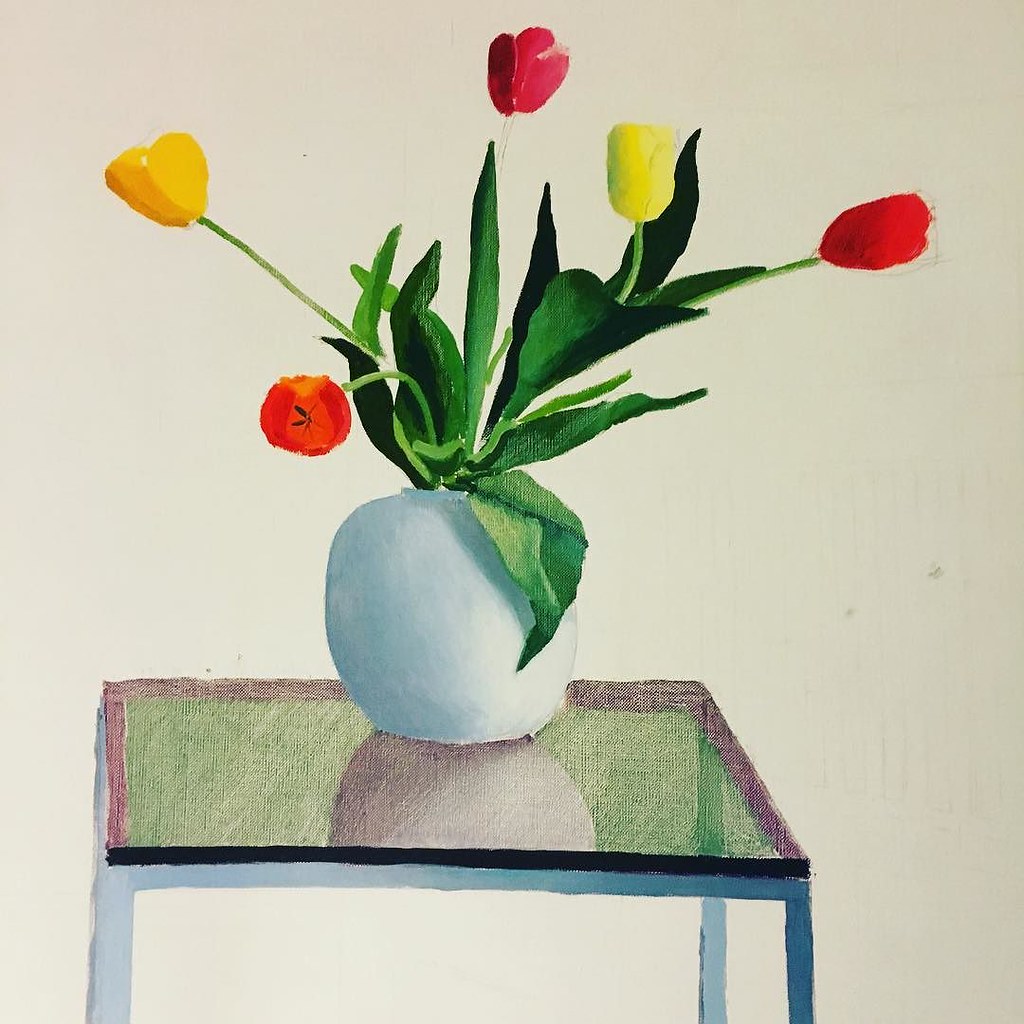This is a detailed color illustration that appears to be created with a combination of paint and color pencils. It portrays a hand-painted scene featuring a square-shaped table with a reflective glass tabletop that has a very light green tint. The table has slightly darker blue legs and a white frame. Situated on the glass surface is a circular white vase. The vase contains five tulips with long, light green stems and large green leaves. The tulips are colored in yellow, pinkish-red, red, and an orangey-red hue. The reflection of the vase on the glass tabletop is clearly visible. The background of the painting is a very light baby blue, enhancing the vivid colors of the tulips and the serene setting. The artwork showcases excellent shading and a harmonious blend of colors, leveraging its reflective elements to add depth and realism.